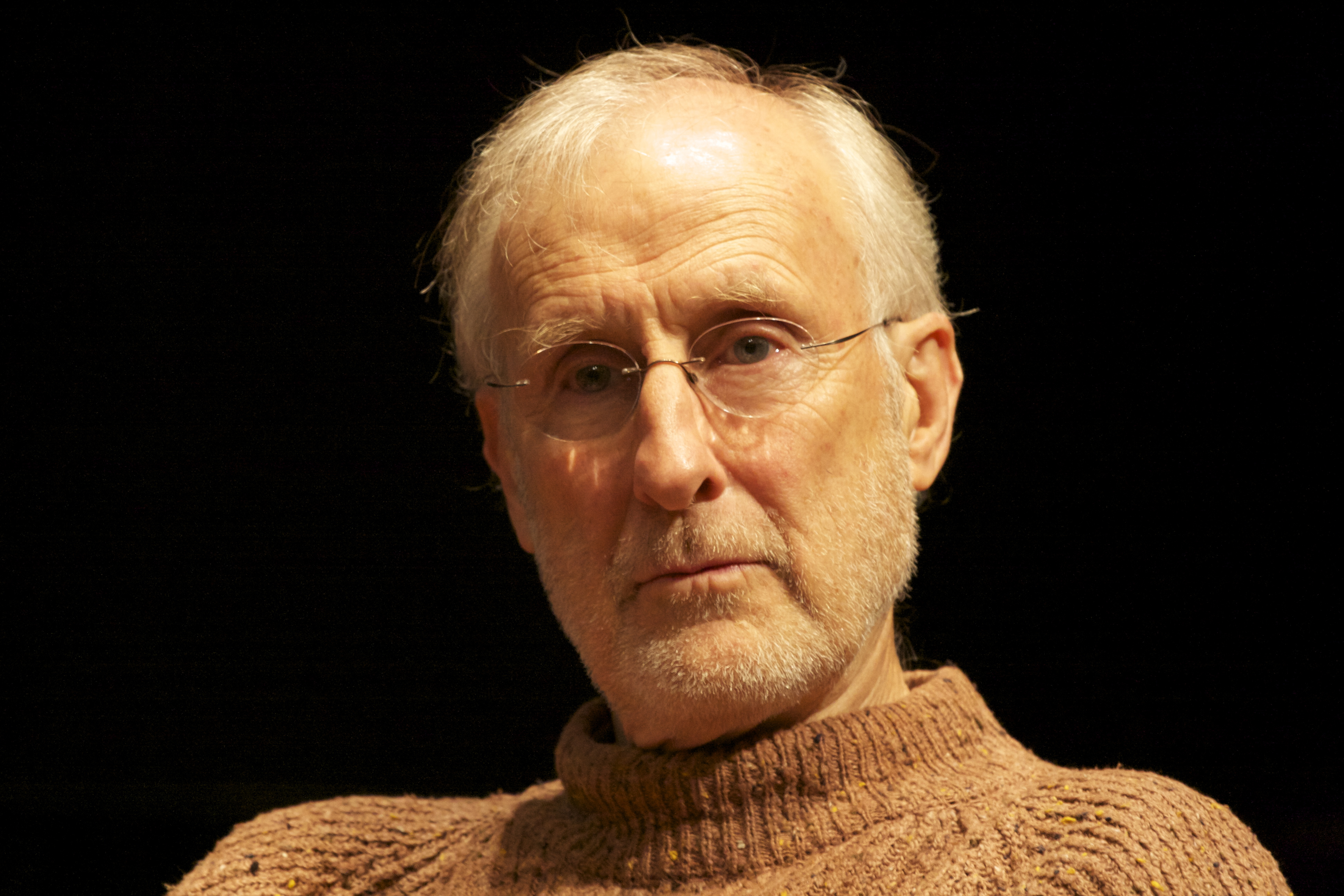This photograph features an older man, potentially in his seventies, set against a pitch-black background. He is dressed in a tannish, possibly speckled sweater with a high collar, resembling a half turtleneck. His attire, paired with his general demeanor, suggests a somber or contemplative mood. The man has a closely cropped gray beard and mustache and sports rimless eyeglasses with straight stems. His gray, wispy hair reveals a significant bald spot, and his bushy, gray eyebrows underline a fairly wrinkled forehead. His blue eyes are visible through the thin-rimmed glasses, projecting a feeling of sadness or deep thought. Although he is facing forward, he seems lost in thought rather than engaged with the camera, exuding a serious, reflective aura.